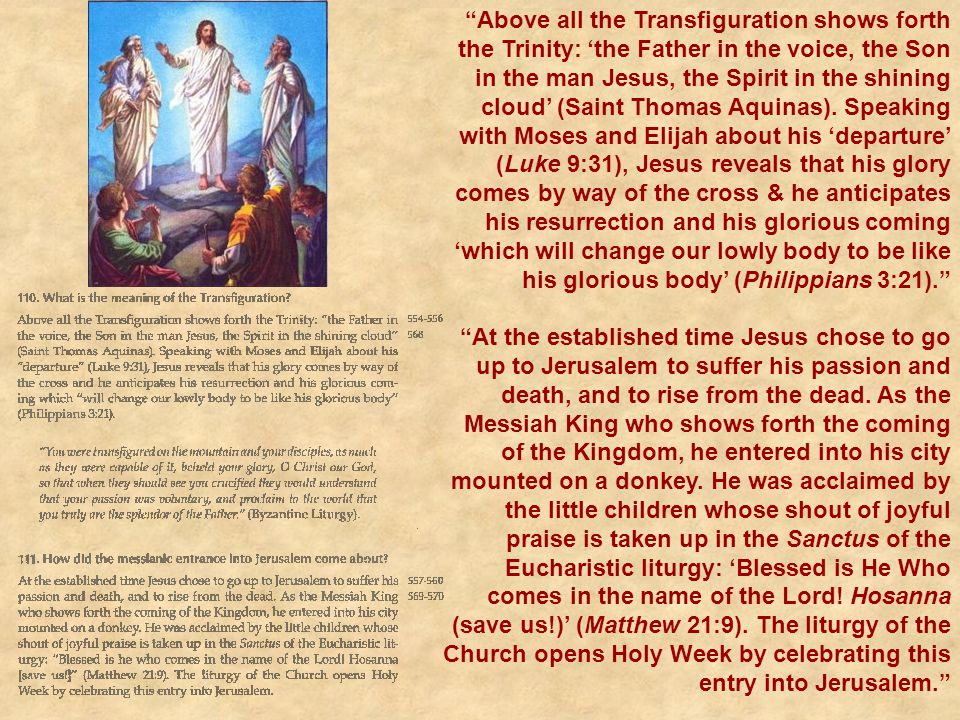The image is a detailed illustration possibly from a religious text, depicting the transfiguration of Jesus on a mountaintop against a backdrop of blue skies with radiant light emanating from behind him. Jesus, adorned in a white toga-like outfit, stands with two men on either side—possibly Moses and Elijah—in various colored garb. Below them, three disciples or apostles are seen from behind, gazing up at the scene. The left corner of the image is captioned with "Number 110, What is the meaning of transfiguration?" followed by two explanatory paragraphs. Another section titled "Number 111, How did the entrance into Jerusalem come about?" is placed beneath, with a subsequent paragraph explaining the event. To the right, the layout includes two paragraphs in a larger red font; one prominently begins with "Above all the transfiguration shows forth the Trinity..." expounding theological interpretations with biblical references. The whole image has a light tan or beige background, enhancing the structured, infographic-like format.